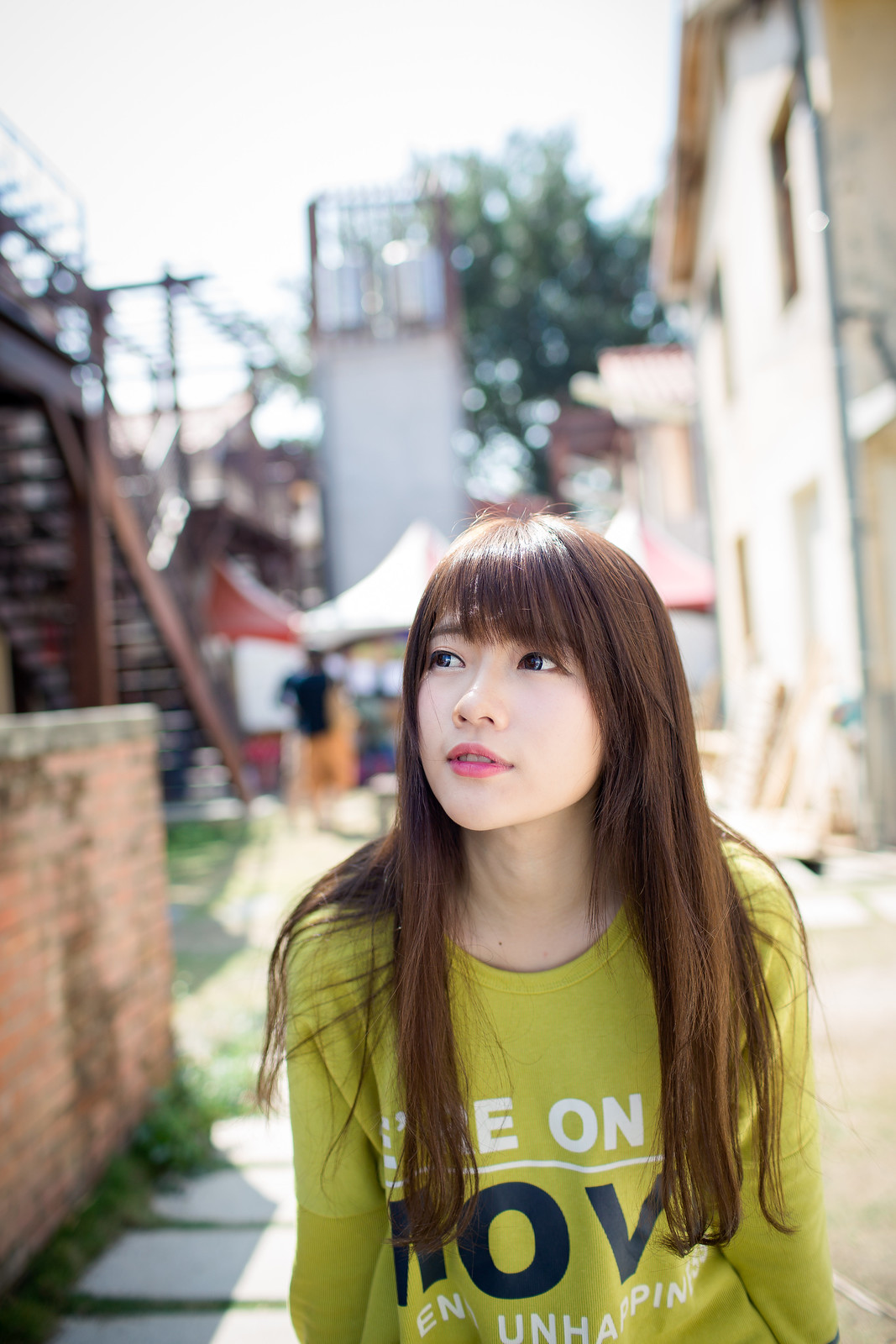In this detailed photograph, a young Asian woman with long brown hair and pink lipstick is centrally positioned, gazing thoughtfully to her left. She is wearing a green long-sleeve crew neck shirt with partially obscured text. The letters on her shirt read "E-E-O-N" in white, "M-O-V" in black, and "END UNHAPPINESS" in white. The setting appears to be outdoors in the middle of the day, possibly in a downtown area. Behind her, the background is blurred, highlighting her as the main focus. Nonetheless, the visible elements include several structures, such as multiple pavilions with tent tops, a rusted scaffolding and metal stairs on the left, a stone road to the right, a brick wall to the left, and a concrete building. There are also a few people walking in the background, a stone walkway with grass growing between the tiles, and a glimpse of the sky at the top of the image. The scene is vividly colorful with shades of tan, gray, green, brown, off-green, dark blue, pink, purple, red, maroon, and white.